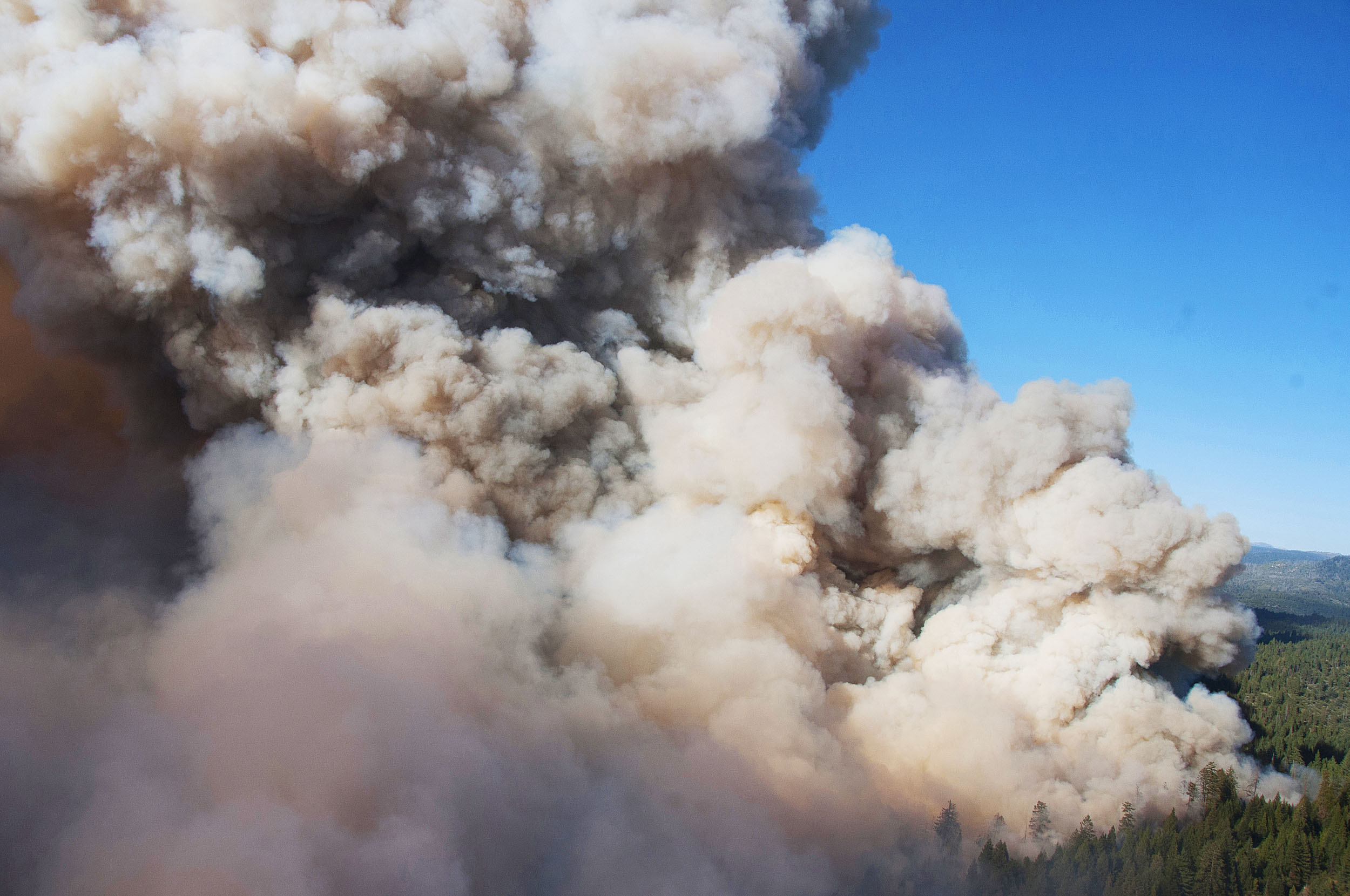This photograph captures an intense and extensive scene of a forest fire. Billows of beige and dark gray smoke dominate almost the entire image, rising from the lower right where the fire is likely located, and being blown towards the left. The thick smoke obscures most of the sky, which paradoxically remains a clear, bright blue in the upper right section, contrasting sharply with the chaotic scene below. At the bottom of the photograph, dense, likely pine trees can be seen, partially engulfed by the thick smoke that appears to be eating them alive. Hints of orange near the base of the smoke strongly suggest active flames, adding to the sense of danger and urgency. On the right side, a portion of what appears to be a forested mountain range is partially visible below the clear sky, providing a stark backdrop to the smoky expanse that dominates the rest of the image.